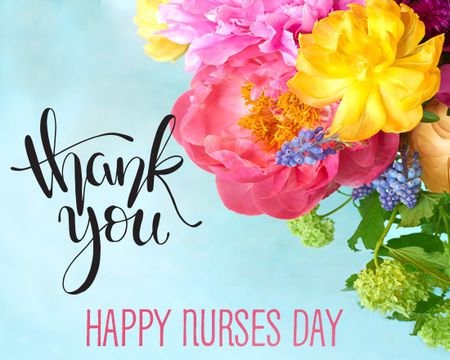This image showcases a thank you card set against a light blue or teal background. The left side features the words "thank you" in elegant black cursive, and below that, in striking red letters, it says "Happy Nurses Day," expressing gratitude for nurses on their special day. On the right side, there's a vibrant bouquet of flowers, which include a variety of blooms such as roses and carnations. The colorful assortment comprises pink, baby pink, hot pink, yellow, and red flowers, along with smaller purple blossoms and greenery. Some flowers have orange centers and yellowish pollen clusters, adding to the rich, detailed presentation. The card appears to be something people might share on social media to celebrate and show appreciation for nurses.